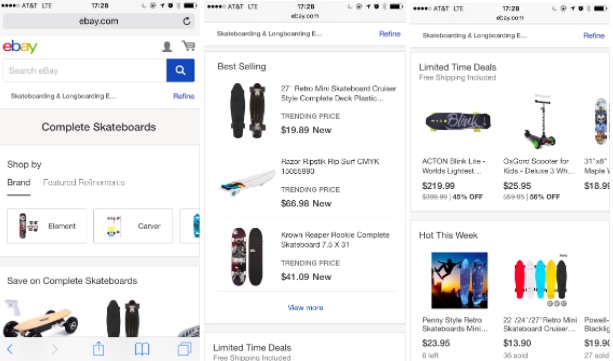This image captures a web page that appears to be an eBay ad focusing on skateboards and skateboarding equipment. The top of the page displays the URL eBay.com, indicating it's an eBay listing, and the AT&T logo suggests the page is accessed via someone's internet or phone provider.

The upper section of the page features a navigation menu, while the focal point displays an array of skateboard listings under various categories. On the left, there's a search result for "complete skateboards," and to the right, highlighted sections include "Best-Selling" and "Limited Time Deals."

The "Best-Selling" section showcases a selection of skateboards, with prices starting from $18 and going up to $219.99. Among these, there's a notable scooter-style board priced at $25.95. Further down, a "Hot This Week" tab lists popular items, featuring blue skateboards at $23.95 and vibrant rainbow-patterned boards at $13.90.

The website features a clean, blue and white aesthetic, with the eBay logo prominently displayed on the top left in its characteristic multi-color design.